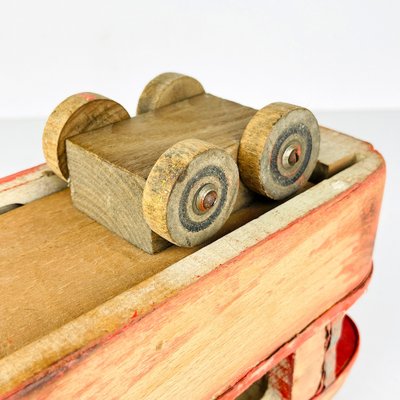The photograph depicts a handcrafted wooden toy car composed of a rectangular unfinished wooden block with four perfectly round wooden wheels, affixed with visible screws or nails. The toy car is turned upside down, revealing the undercarriage and the precise joining of its components. This car rests atop a larger wooden structure, which appears to be a toy as well, distinguished by a reddish stain resembling cherry or redwood. The larger structure features some black scuff marks on the top left side, suggesting possible burn marks. This structure is rectangular and two-tiered, with an interior section painted red, possibly made of cloth, visible at its lower end. Both toys are oriented toward the right, set against a light gray background.